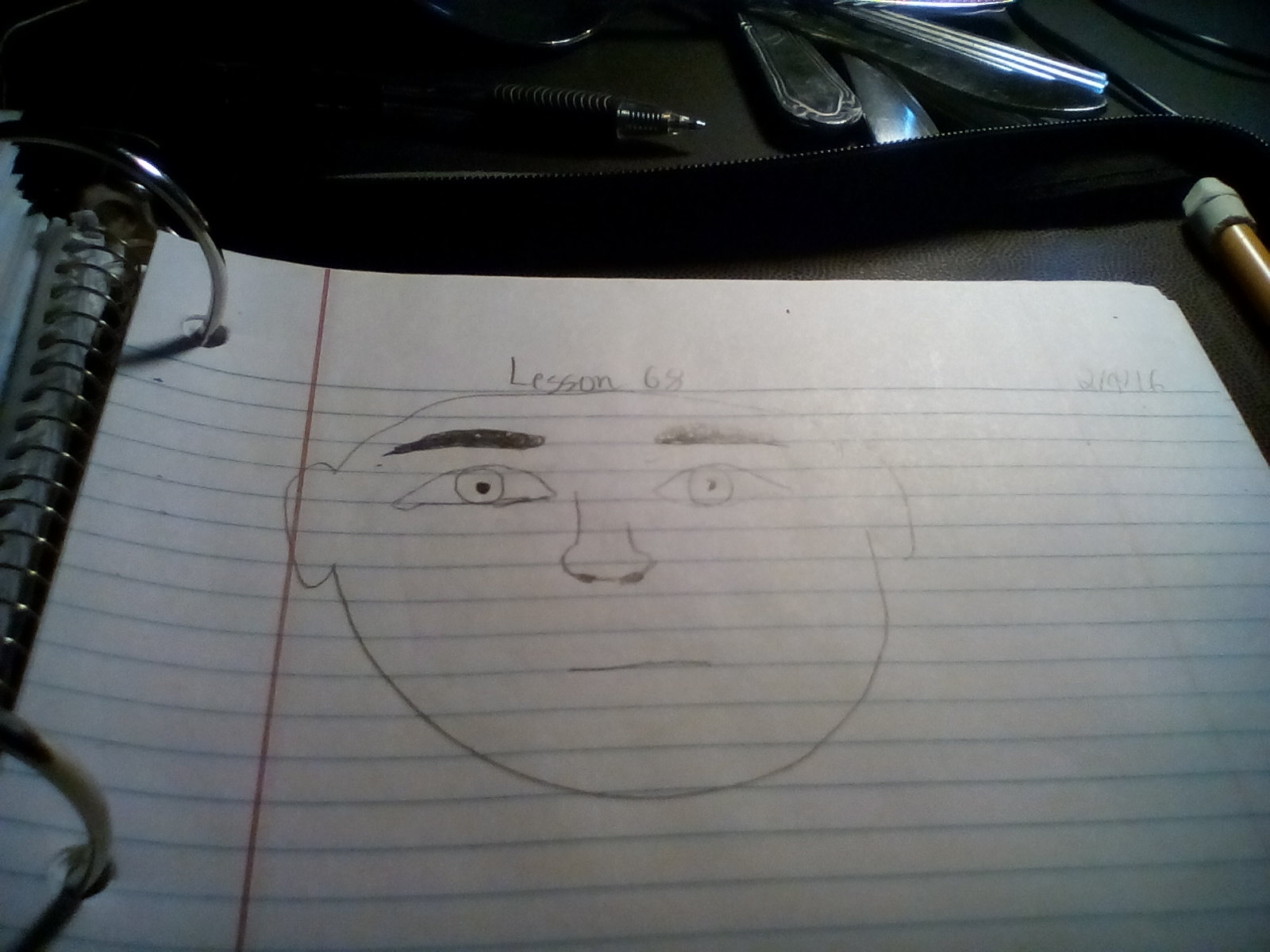This detailed image shows a close-up of a spiral-bound notebook opened to a page of white, blue-lined grid paper. At the top of the page, "Lesson 68" is written, and to the upper right corner, the date "February 9, 2016" is visible. The central feature of the page is a meticulously drawn face with a wide, oval shape. The face is bald, without any hair, and features large, thick black eyebrows that are straight. The eyes are depicted as white circles with small black dots in the center for pupils, surrounded by large eyelids. The nose is simple, with two black circles representing the nostrils, and the mouth is a thin, straight black line with no expression. 

The notebook page, perforated for insertion into the spiral binding, rests on a black surface, which could be a table. Above the notebook on this surface, there is an open black pen and some silverware partially visible. The meticulous detail of the drawing and the neat grid paper format suggest a deliberate and structured approach.